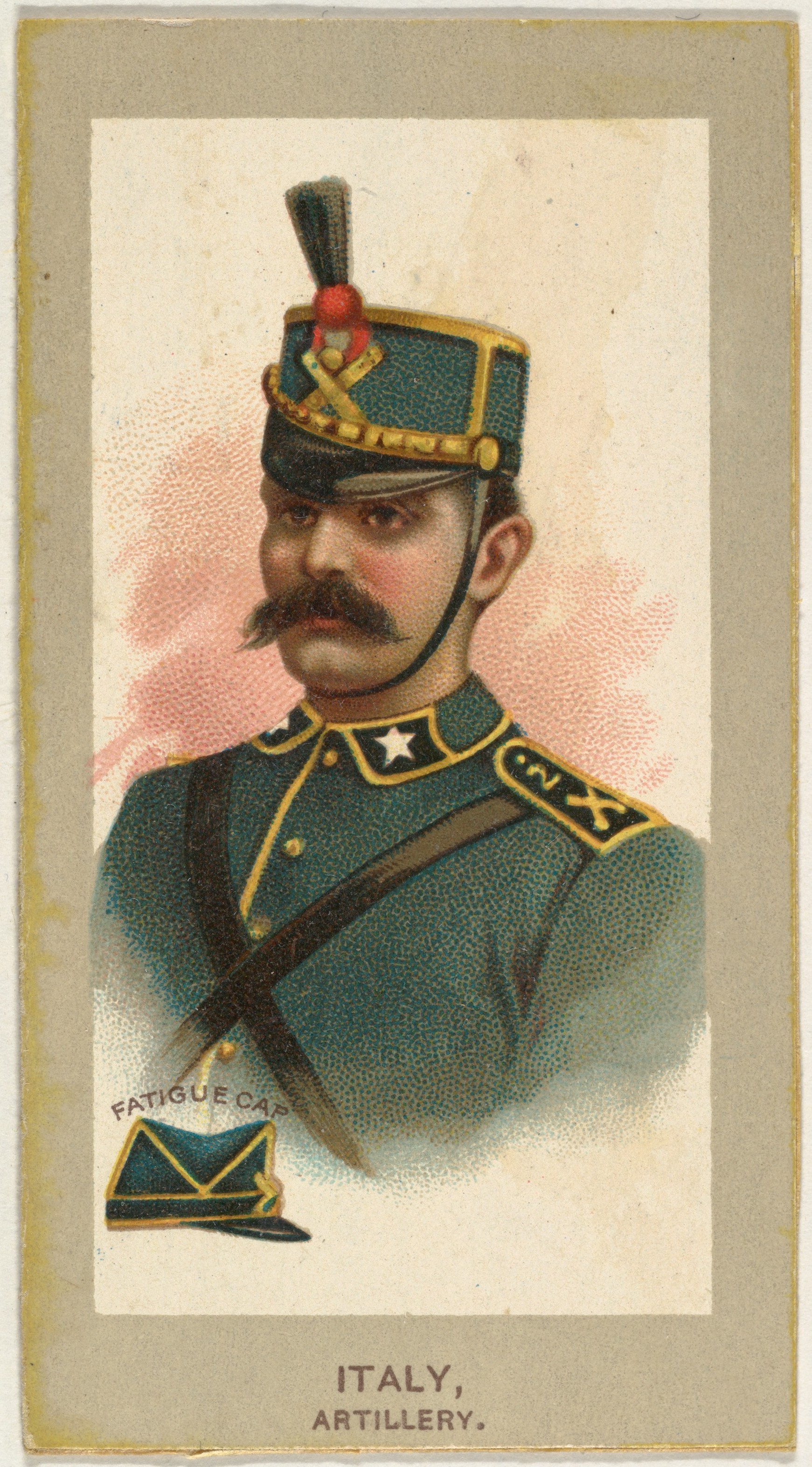This detailed caption combines and refines the descriptions provided. 

The image is a vintage print or drawing depicting an Italian artillery soldier. The label at the bottom of the print reads "Italy Artillery" in a simple all-caps, brown font. The artwork features the soldier in the center, clad in a teal green uniform with gold trim and buttons. He sports a prominent, large, and hairy mustache and has no beard, gazing towards the left with a neutral expression. The soldier wears a distinctive green and gold hat bearing an X symbol on the front, topped with a red and black item, possibly a brush with a red holder. His collars feature two white stars on either side, and black straps form a large X across his chest. The drawing is set against a white backdrop with a pink blush and is framed or matted in taupe gray. There is also text within the image itself, indicating an alternate fatigue cap that the soldier could wear, illustrated in both the foreground and background.